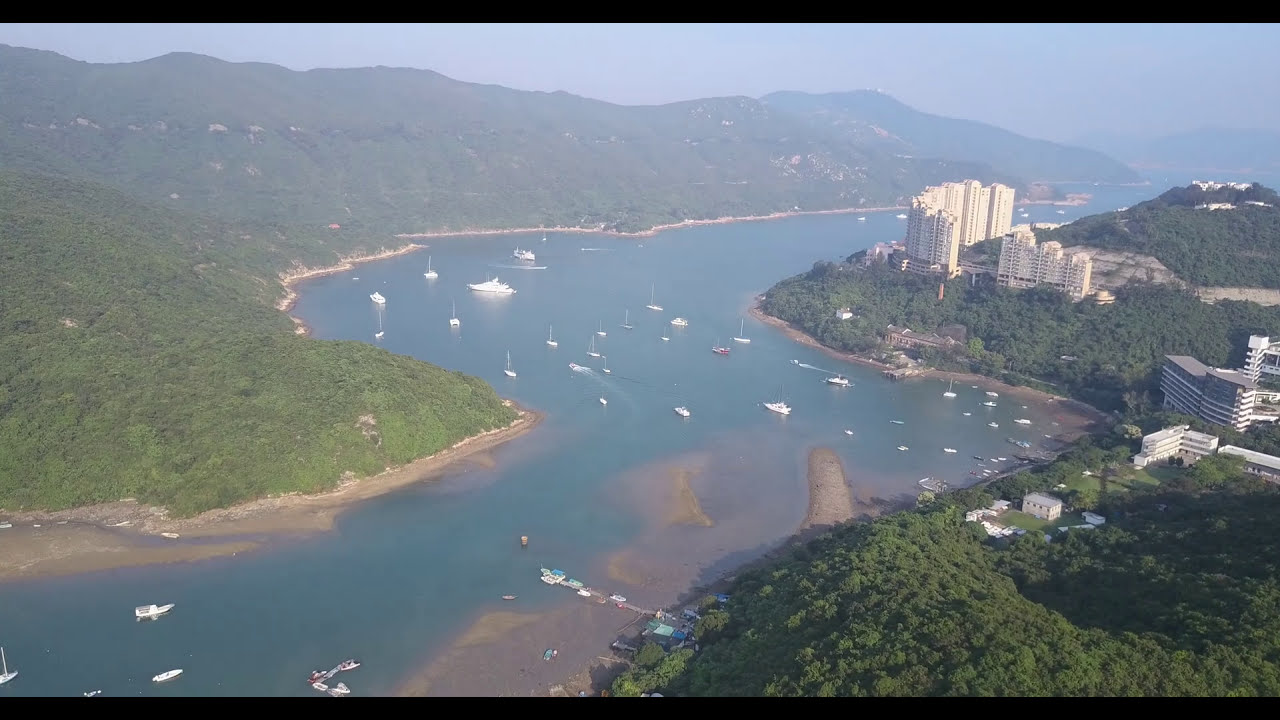The image is an aerial photograph depicting a winding river, which might be an estuary, extending from the bottom left to the top right corner of the frame. The waterway is predominantly blue, merging into darker brown shades near the shorelines. On the right shoreline, lush, bright green trees cover the land, among which are clusters of white buildings, including a notably tall high-rise structure possibly serving as a hotel. Additionally, there are other significant white buildings and a smaller two-story white building, surrounded by trees. Along the left side of the river, the landscape consists solely of dense green hills dotted with low trees, devoid of any built structures. The river itself is adorned with an array of boats, primarily white with a few red ones, and several small docks from which these boats are moored. Thin black lines border the image at the top and bottom, framing the scenic outdoor view of this vibrant and bustling natural and man-made landscape.